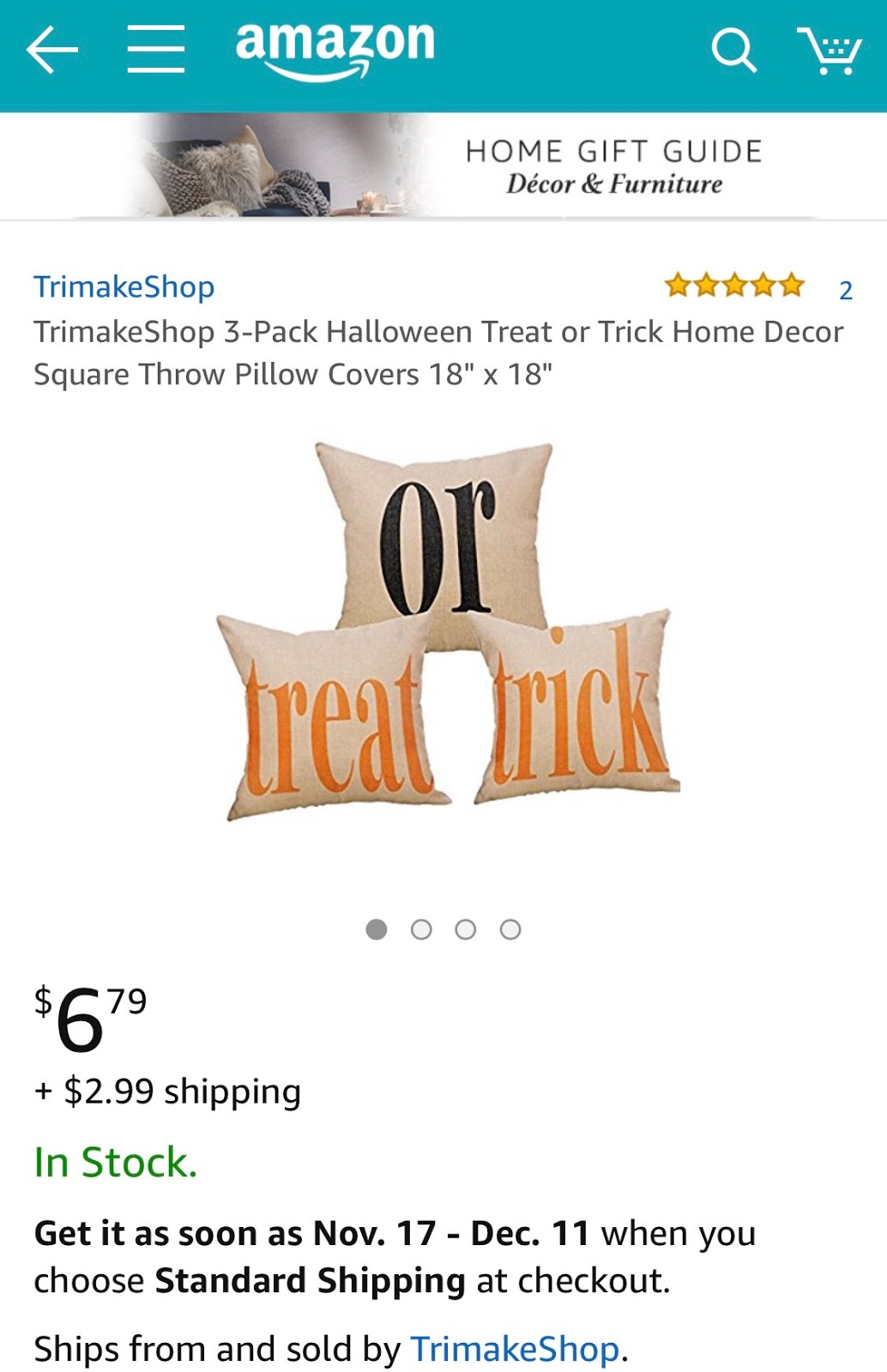This is an image of a three-pack Halloween-themed decorative pillow set by Trimake Shop available on Amazon. The pillows, measuring 18x18 inches, feature phrases like "Trick or Treat." The product has garnered two five-star reviews so far. 

The image is framed within the familiar Amazon interface, showcasing the white Amazon logo with the signature swoosh arrow at the top. Navigation elements such as the back button, a three-line menu icon, a magnifying glass for search, and a shopping cart icon displaying the number of items in the cart, are visible.

Below the product images, the price is listed as $6.79 plus $2.99 for shipping. The current stock status is highlighted in green, and it notes that if ordered now, the item will arrive between November 17th and December 11th with standard shipping. 

The product is sold by and ships from Trimake Shop. This is one of four images available, as indicated by the dots below the current image (image 1 of 4).

Additionally, a banner between the product rating and the Amazon logo at the top showcases a cozy living room scene with pillows and blankets, promoting the "Home Gift Guide" with the words "Decor and Furniture" italicized and bolded.